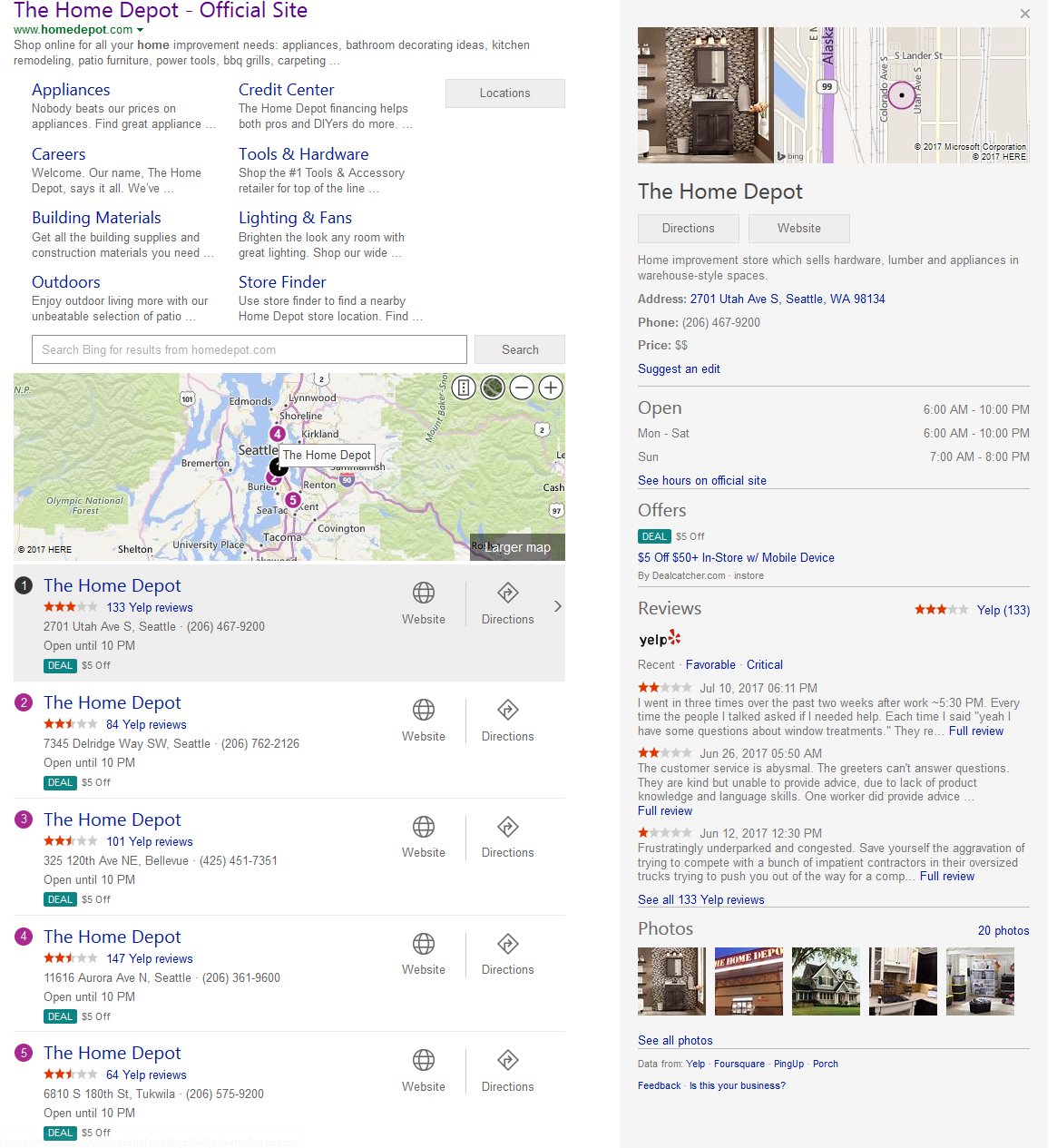This image is a detailed snapshot of the official Home Depot website. At the top, the URL "www.homedepot.com" confirms the authenticity of the site. Below the main navigation bar, several categories are visible, including Appliances, Careers, Building Materials, Outdoors, Credit Center, Tools & Hardware, Lighting & Fans, and Store Finder.

Further down, a map is displayed, focusing on Seattle, Washington, pinpointing the exact locations of various Home Depot stores. Each pin provides details such as store ratings, Yelp reviews, links to the store's website, and navigation directions.

Prominently showcased is the Home Depot’s logo, alongside hyperlinks offering directions and access to their website. An advertisement highlights a promotional offer of $5 off a $50 purchase.

Scrolling down, user reviews from Yelp are presented. One particular review stands out, where a customer rated the store two stars, commenting on their repeated attempts to obtain assistance with window treatments after work at 5:30 PM. The incomplete review invites viewers to read the full commentary by following the provided link. 

This carefully arranged webpage guides users effortlessly through the navigation and provides essential resources at a glance.